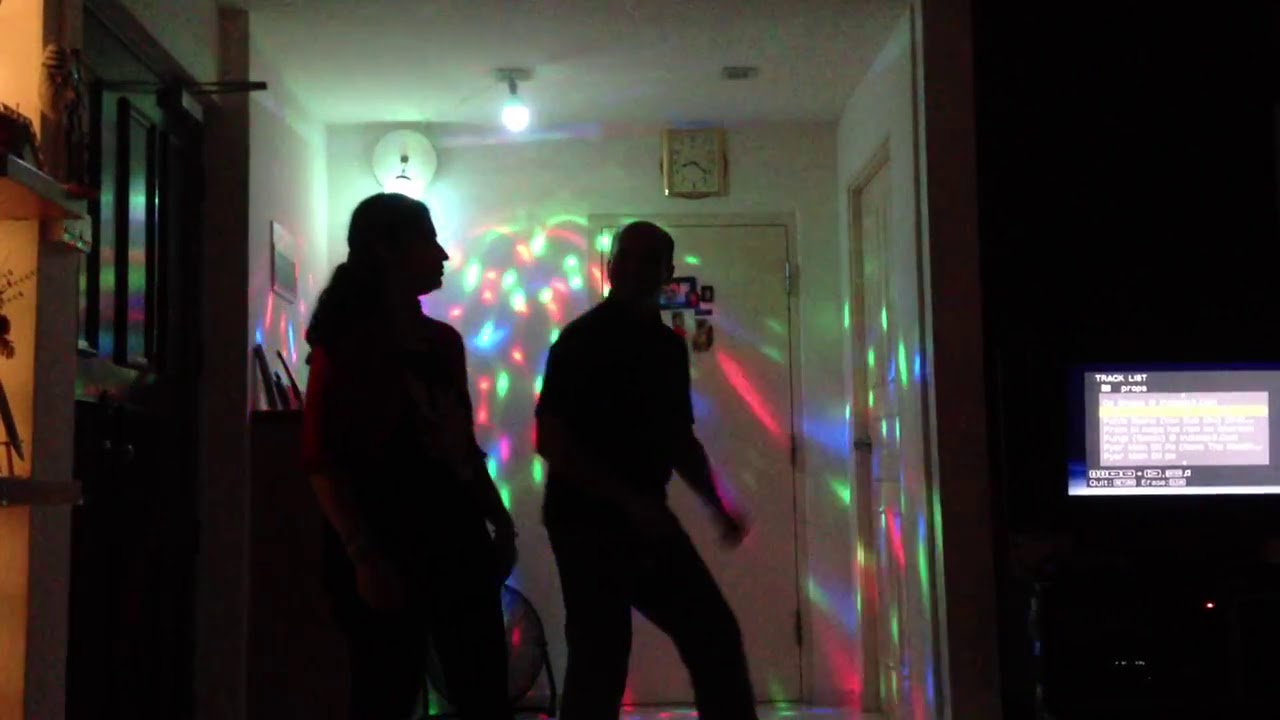The photo is a color, landscape-oriented image capturing the silhouettes of a man and a woman dancing at night in a dimly lit apartment. The scene is backlit, causing the dancers to appear as dark figures without clear facial features, adding a sense of mystery. They are positioned against a white wall illuminated by multicolored lights, reminiscent of a disco ball effect. The man is slightly bent over facing the right, while the woman stands with her head tilted back, and they seem to be looking at each other. Overhead, a single light bulb provides minimal illumination, accompanied by a small rectangular clock above a door that reads 8:20. The right side of the image features a dark room with an open laptop displaying the words "TRACK LIST," suggesting music is playing. The apartment has additional doors and shelves, and framed photos are visible on a brown wall to the left. The overall style of the photograph is representational realism.